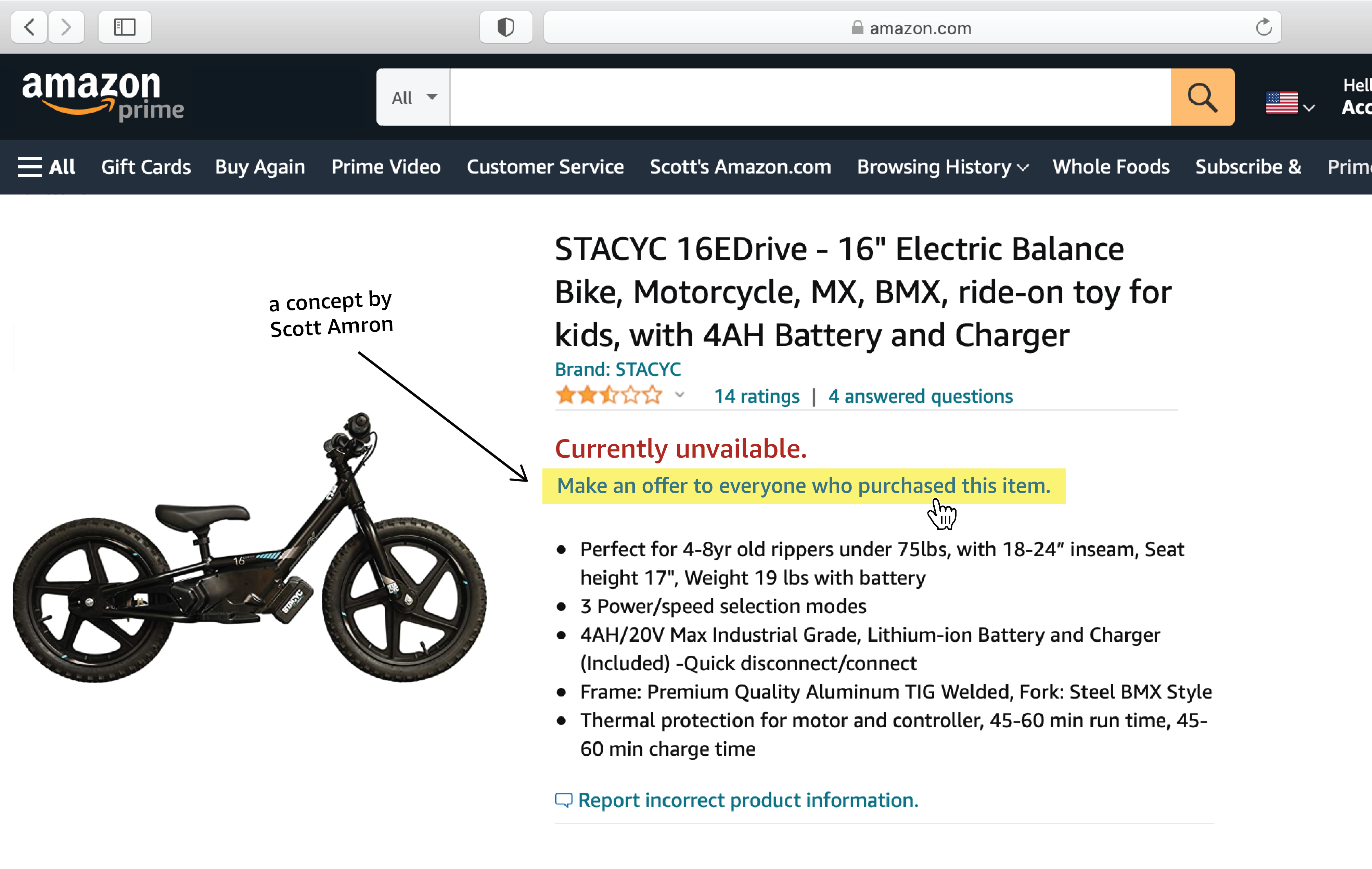The image is a screenshot of an Amazon product page featuring a black electric motorcycle designed for children. The page has a clean white background, prominently displaying the product named "STACYC 16eDrive 16" Electric Balance Bike." The motorcycle is oriented with the handlebars to the right and the seat to the left.

The product description details the following features:
- Intended for children aged 4 to 8 years, weighing under 75 pounds and with an inseam between 18 to 24 inches.
- Seat height is 17 inches, and the bike weighs 19 pounds including the battery.
- Equipped with a 4AH, 20V max industrial-grade lithium-ion battery and charger.
- Offers three power speed selection modes and a quick disconnect/connect feature for the battery.
- Built with a premium quality aluminum TIG welded frame and a steel BMX-style fork.
- Provides thermal protection for both the motor and controller.
- The battery allows for 45 to 60 minutes of runtime and takes the same amount of time to charge fully.

The page indicates that the product has only 14 customer ratings, averaging a two-and-a-half-star rating, and has four answered questions. Currently, the product is listed as unavailable. An additional note mentions a feature allowing users to "make an offer to everyone who purchased this item," conceptualized by Scott Amron. There's also an option to report any incorrect product information.

Overall, the Amazon page offers a detailed view of the children's electric motorcycle, including its specifications, user feedback, and availability status.